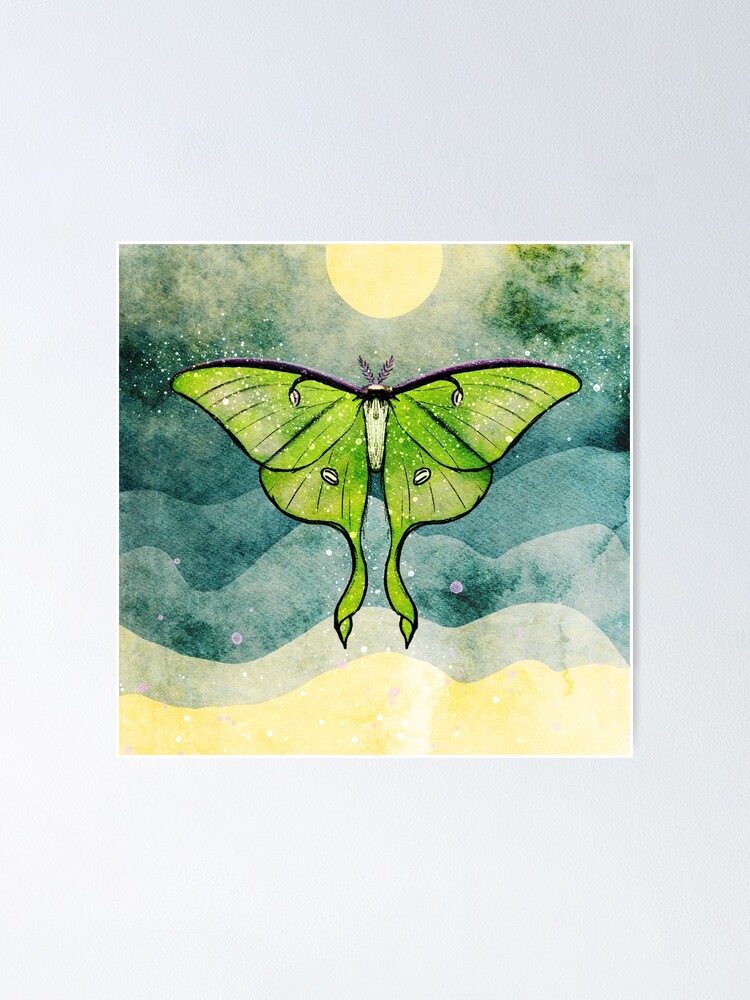This detailed and romantic watercolor painting, hanging on a white wall and framed with a thin white border, depicts an abstract and dreamy green moth or butterfly flying upward towards the moon. The piece is set against a vibrant backdrop that transitions from yellow at the bottom to darker shades of blue at the top, resembling layered ocean waves. These layered waves are drawn without outlines, using soft transitions that suggest the ethereal quality of watercolor. At the very top, a bright circular moon is partially visible, illuminating the night sky and surrounded by light greens and blues, adding to the painting's whimsical feel. The moth itself, outlined boldly, contrasts with the background and appears to leave behind a trail of magical dust, enhancing its otherworldly appearance. The overall composition evokes a sense of free-flowing movement and fantasy, with the moth's abstract, almost fabric-like texture contributing to a gentle and romantic aesthetic.